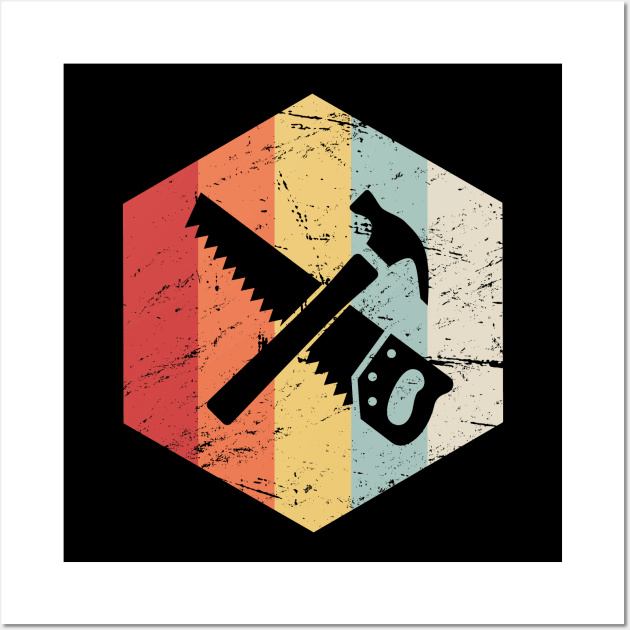The image showcases a logo or design, possibly for a construction company, featuring a black square set against a white background with a blue outline framing the square. Inside the black square, there is a hexagon with six sides that contains five vertical stripes in red, orange, yellow, light blue, and white, from left to right. Black lines create texture and shading across these colorful stripes.

At the center of the hexagon, a hammer and a hand saw intersect in an X shape, depicted as shadowy silhouettes. The hammer, with its handle stylistically separated from the metal part, is positioned with its claw directed downward towards the lower right corner. The saw, with exaggerated teeth and a handle distinctly separated from its blade, has three holes where the handle meets the blade, and it points diagonally to the upper left. The overall image lacks any text or advertisement, adding to its abstract yet industrial aesthetic, suggesting it could represent a construction-related business.